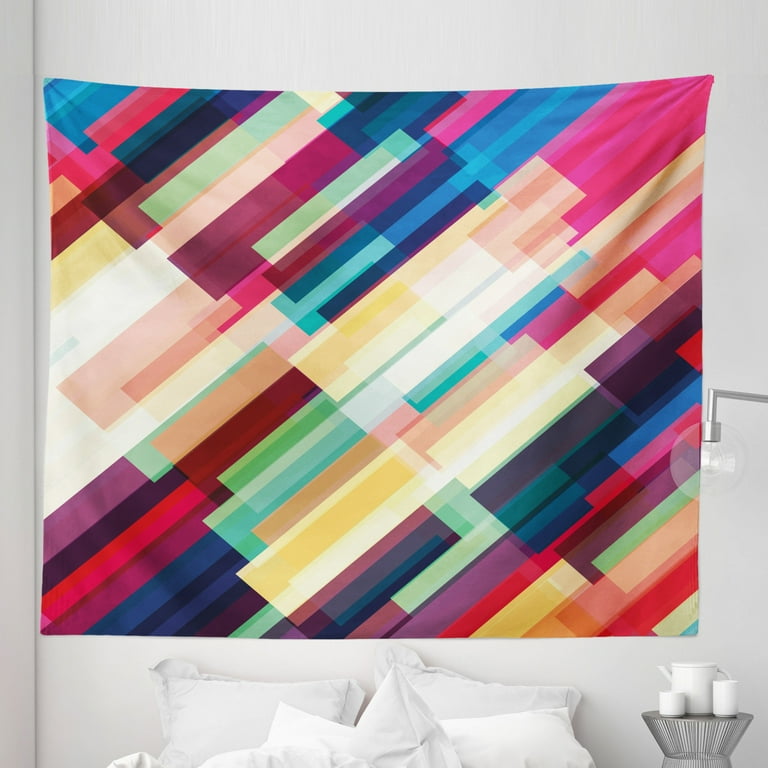This photo captures a minimalist bedroom adorned with a distinctive, avant-garde wall hanging above the bed. The bedroom features stark white bedding, including white sheets, pillows, and pillowcases, contributing to its monochromatic theme. A metal nightstand sits beside the bed, holding a white water pitcher, cup, and tumbler. Above the nightstand, a brushed nickel spotlight lamp illuminates the scene with a soft glow. The focal point of the room is a vibrant, multi-colored hanging composed of diagonal, rectangular pieces of material, resembling a dynamic, abstract quilt. The hanging stretches from the upper right to the lower left of the image, showcasing a rich array of colors including deep pink, blue, dark blue, light blue, green, yellow, red, brown, white, and various other shades. This stunning piece, tacked up on the wall, injects a lively burst of color into the otherwise neutral palette of the bedroom.